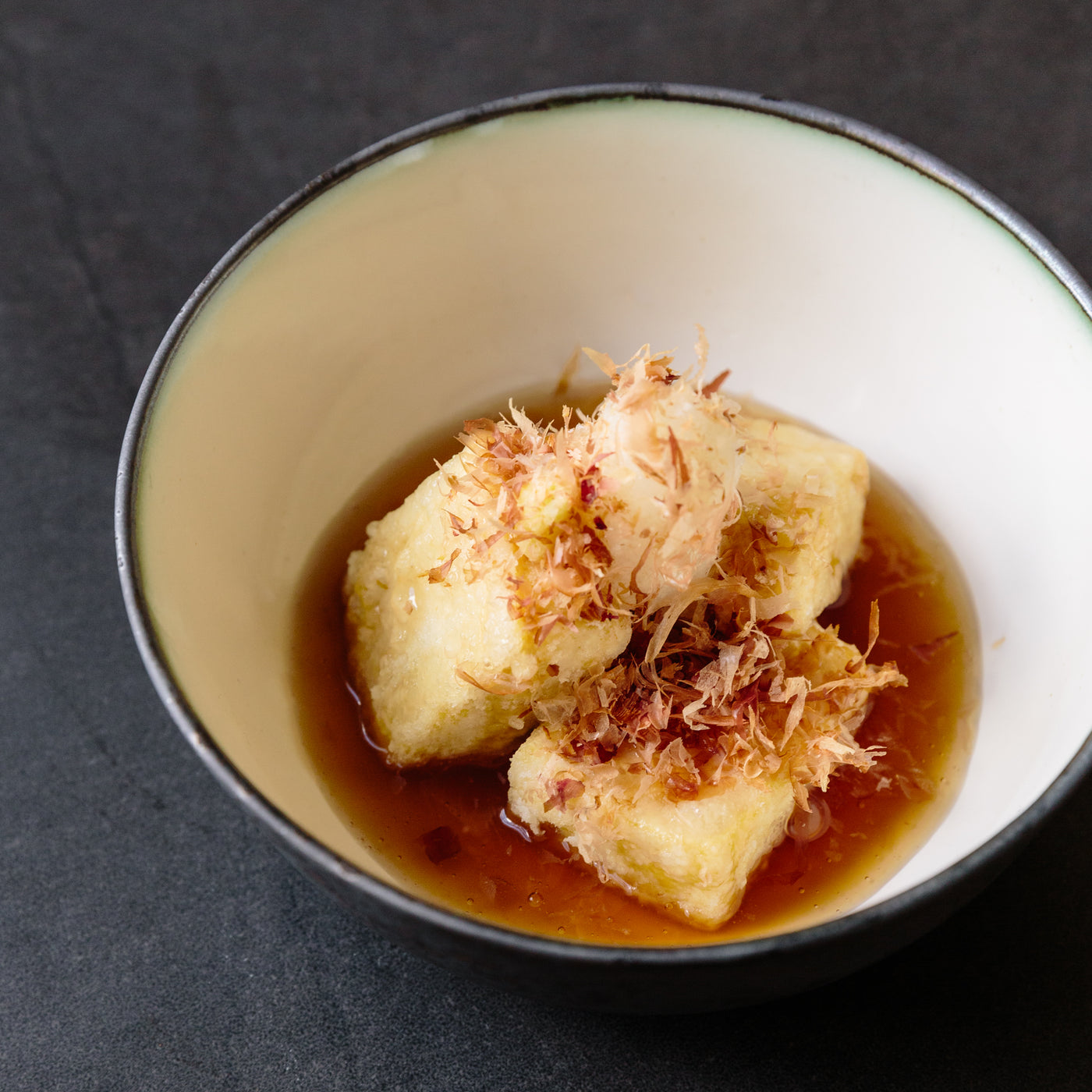This photo captures a meticulous presentation of a culinary dish set against a solid charcoal gray background. The focal point is a white ceramic bowl with a distinctive shimmery silver rim. Positioned at an overhead angle, the bowl reveals a beautifully arranged trio of cooked tofu squares nestled in a golden-brown sauce at the bottom. Each tofu piece is meticulously topped with light brown slivers of crispy tuna, adding texture and contrast. Speckled throughout the sauce are various flecks and strands, possibly resembling toasted coconut or daikon radish, enhancing the visual and textural complexity of the dish.